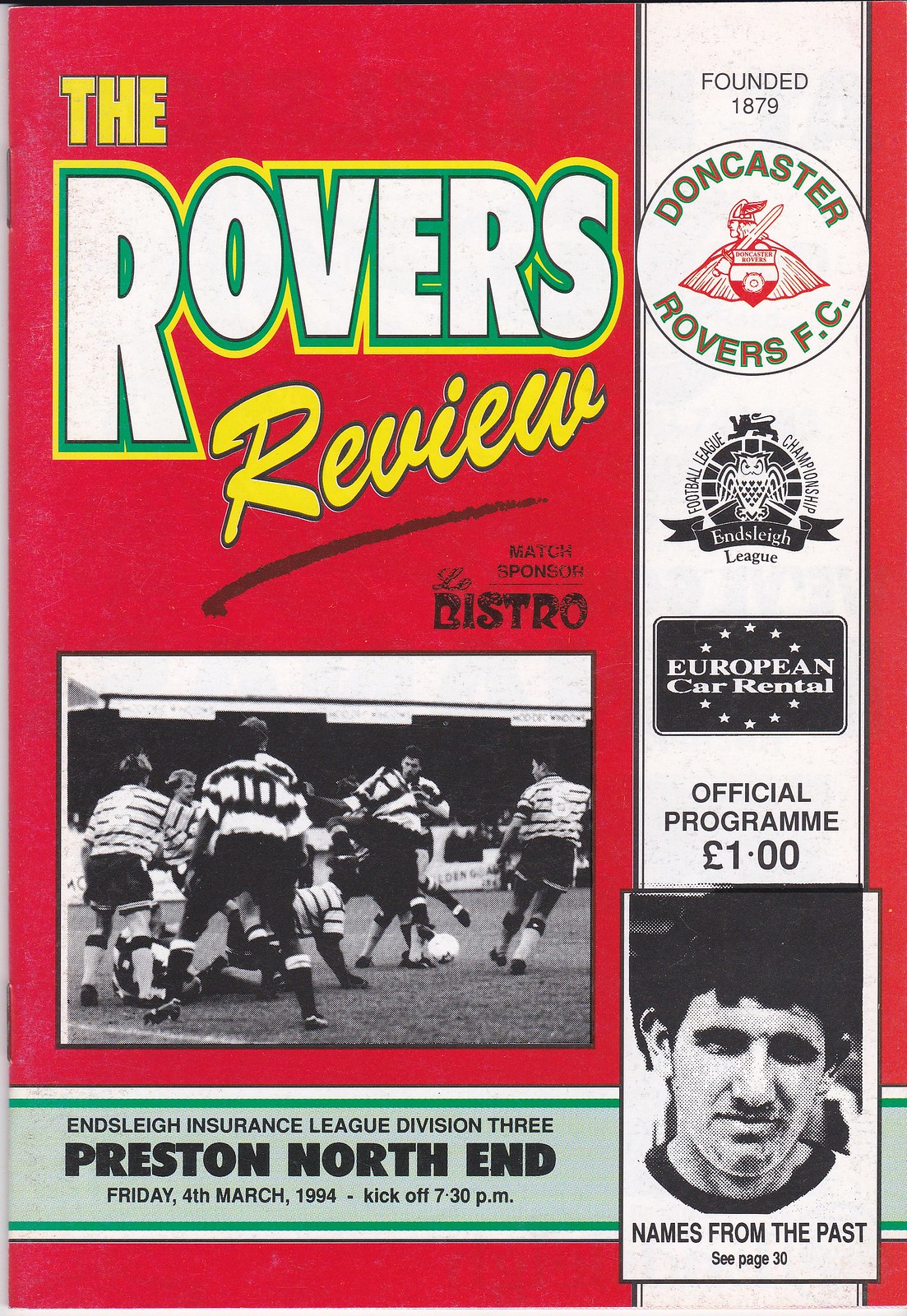The cover of this football program, titled "The Rovers Review," prominently features the match sponsor, Le Bistro, set against a red background. Below this, a black-and-white action photograph captures players battling for the ball on the field. The program is for an Ensley Insurance League Division III match between Preston North End and Doncaster Rovers FC, scheduled for Friday, March 4, 1994, with a kickoff at 7.30 p.m., as stated on a green banner at the bottom. To the right, there is a vertical section highlighting that Doncaster Rovers FC was founded in 1879, with the Football League Championship logo and an advertisement for European Car Rental below it. The program is priced at £1. Additionally, a headshot of a man labelled "Names from the Past" directs readers to page 30 for more information.